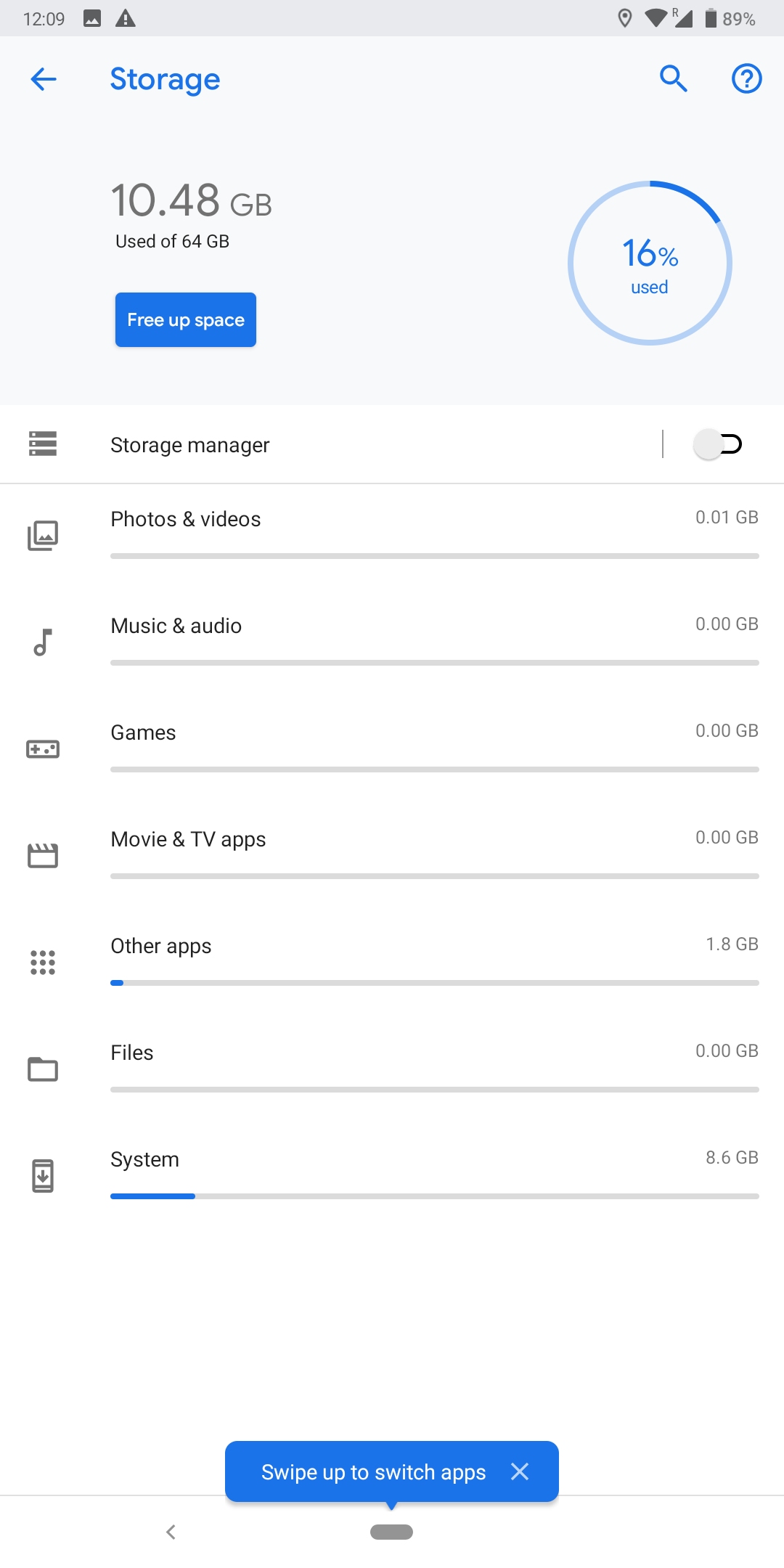The image captures a phone screen displaying a storage management interface. 

At the top, there's a "Back" button on the left side, which heads back to the previous screen. Next to it, the title "Storage and Blueprint" is prominently displayed. On the right side, there is a blue magnifying glass icon followed by a blue question mark enclosed in a blue circle. Below this header, it reads "10.48 GB used of 64 GB," with further information indicating "16% used." To the right, there’s a visually represented circular graph, where a small segment at the top is filled in blue, contrasted against the rest, which is light blue.

Further down, there’s a blue link labeled "Free Up Space" located towards the bottom left. Below this, several categories are listed under "Storage Manager":
- **Photos and Videos**: 0.01 GB
- **Music and Audio**: 0.00 GB
- **Games**: 0.00 GB
- **Movies and TV apps**: 0.00 GB
- **Other apps**: 1.8 GB
- **Files**: 0.00 GB
- **System**: 8.6 GB

"Storage Manager" has a lock icon at the end, suggesting restricted access or a need for authentication. Towards the bottom of the screen, there is an actionable box labeled "Swipe up to switch apps."